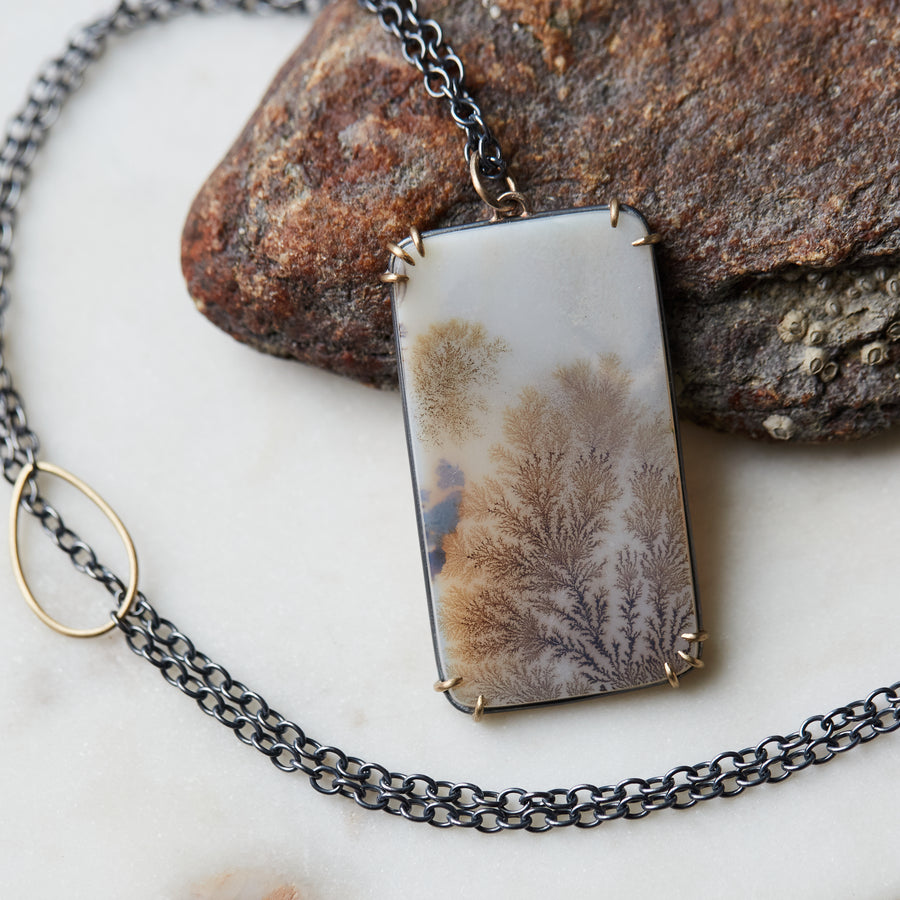The image is a high-quality, top-down photograph showcasing a necklace elegantly displayed against a large, reddish-brown stone with dark gray to black accents. The necklace features a dark gray to black metal chain with a rectangular moss agate pendant that is notably eye-catching. The moss agate is characterized by its opaque white base interspersed with intricate brown and tan mineral tendrils, resembling tree branches reaching through a misty forest. Securely fastened at the corners by gold prongs, the pendant also includes a gold loop attachment. This combination of earth-toned elements complements the natural, organic beauty of the pendant, though the chain appears slightly less remarkable in comparison to the exquisite pendant it supports.